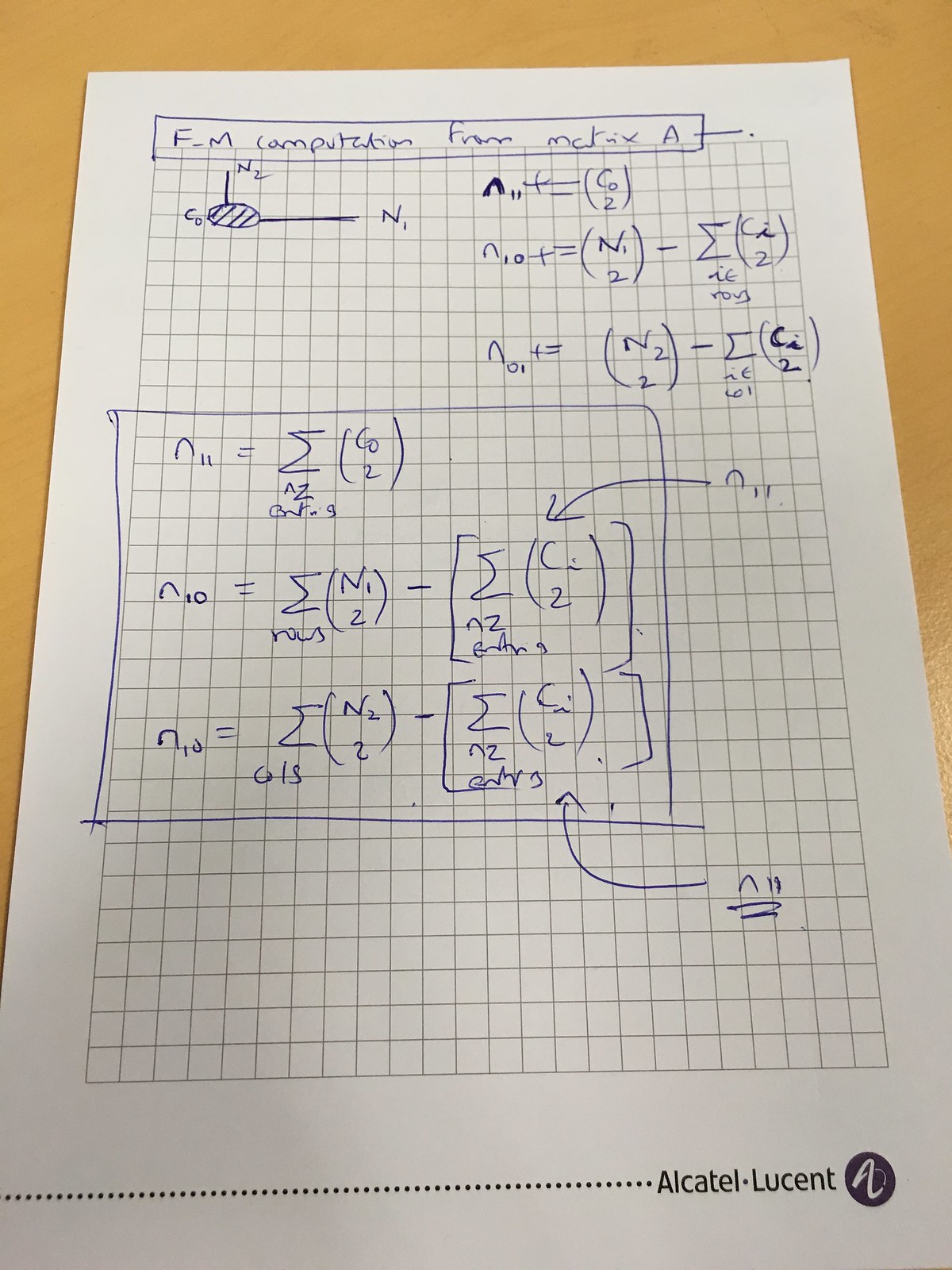In this detailed photograph, we observe an oblong sheet of pristine white graph paper adorned with various mathematical annotations. The graph paper is situated on a light brown surface, likely a wooden table. In the lower right-hand corner of the sheet, the name "Alcatel-Lucent" is prominently displayed alongside the company's logo—a circle containing a distinct white letter "A."

At the top of the paper, there's a headline written by hand, though it's difficult to decipher due to the mixed use of block letters and cursive script. Just below this headline, on the right side, reside three equations aligned vertically, likely indicating advanced calculations, possibly from calculus or algebra.

In the center of the paper lies a prominent square, meticulously drawn. To the left of this square, three more equations are inscribed in dark blue ink. Additionally, two other equations are situated on the lower right corner inside the square, stacked one above the other.

Around the square, further annotations are evident. At the top left of the square, there is text, though its precise contents are not readable. This text is accompanied by an arrow pointing towards the equations within the square. Similarly, at the bottom of the square, more handwritten notes accompany another arrow pointing towards the equations, indicating further elaboration or explanation.

The detailed annotations, coupled with the clear corporate branding, suggest that this sheet might encapsulate a complex problem-solving process or a set of instructions possibly related to telecommunications or advanced mathematical analysis.